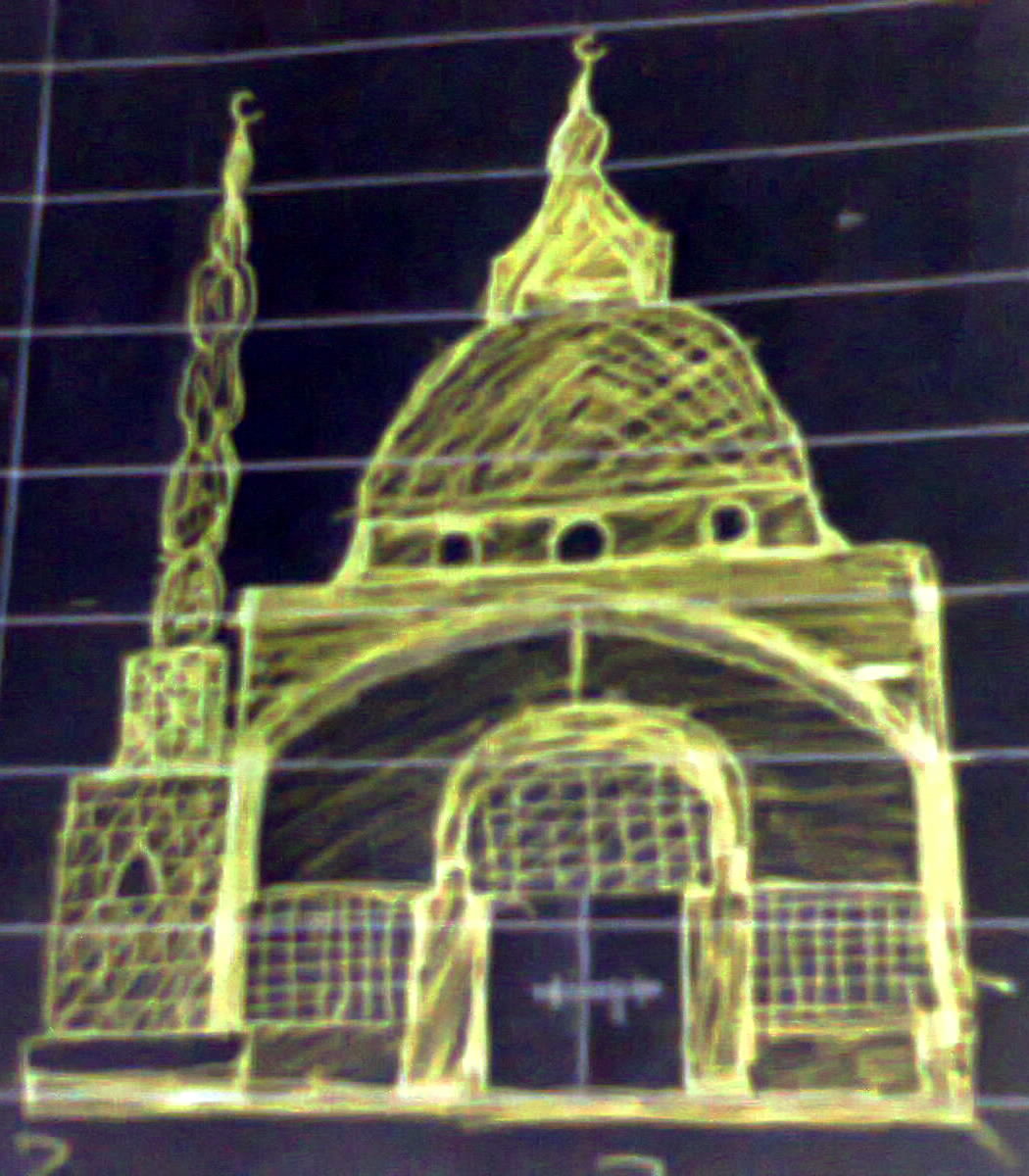In this image, a mosque is intricately depicted using yellow chalk on a blackboard, which has white lines running through it. The mosque features a prominent archway that serves as the main pathway. To the left of the arch, there is a spire, and another spire is positioned on top of the structure. Both spires are adorned with crescent moon symbols. At the center of the arched opening is a doorway with two large black doors secured by a bolted lock. Flanking this doorway are two windows, one on each side, adding to the architectural detail of the scene.